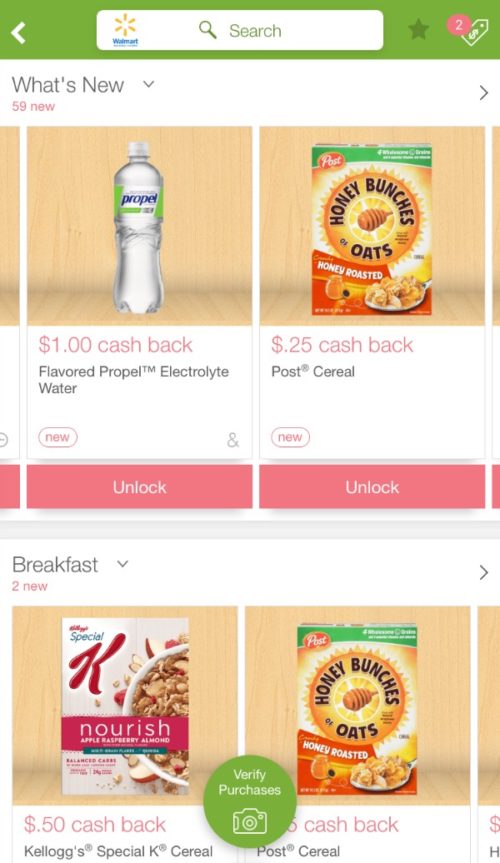This screenshot from Walmart's app features a variety of shopping options and promotions. At the top, there is a search bar adorned with the Walmart icon and a magnifying glass. To the left, a green star on a lighter green header is visible next to an icon of a price tag with the number 2 displayed in an orange oval.

Below the search bar is a subheader labeled "What's New," featuring 59 new items. This section presents a row of pictures showcasing two different products. On the left, there is an image of flavored Propel electrolyte water, which offers $1 cashback, as indicated beneath the product image. To the right, we see a box of Honey Bunches of Oats cereal, which comes with a $25 cashback offer, specified below the image as a Post cereal product. Both items feature an option to unlock cashback offers below at the bottom of their respective images.

Further down, the next subheader titled "Breakfast. Two New." displays two breakfast cereal options. The first is a box of Special K Nourish cereal with a $0.50 cashback offer, branded as Kellogg's Special K cereal. Next to it is another image of Honey Bunches of Oats cereal, although the cashback amount is obscured by a green oval. This section also includes a prompt to verify purchases with a camera. Below the image, it additionally specifies the Honey Bunches of Oats product as a Post cereal.